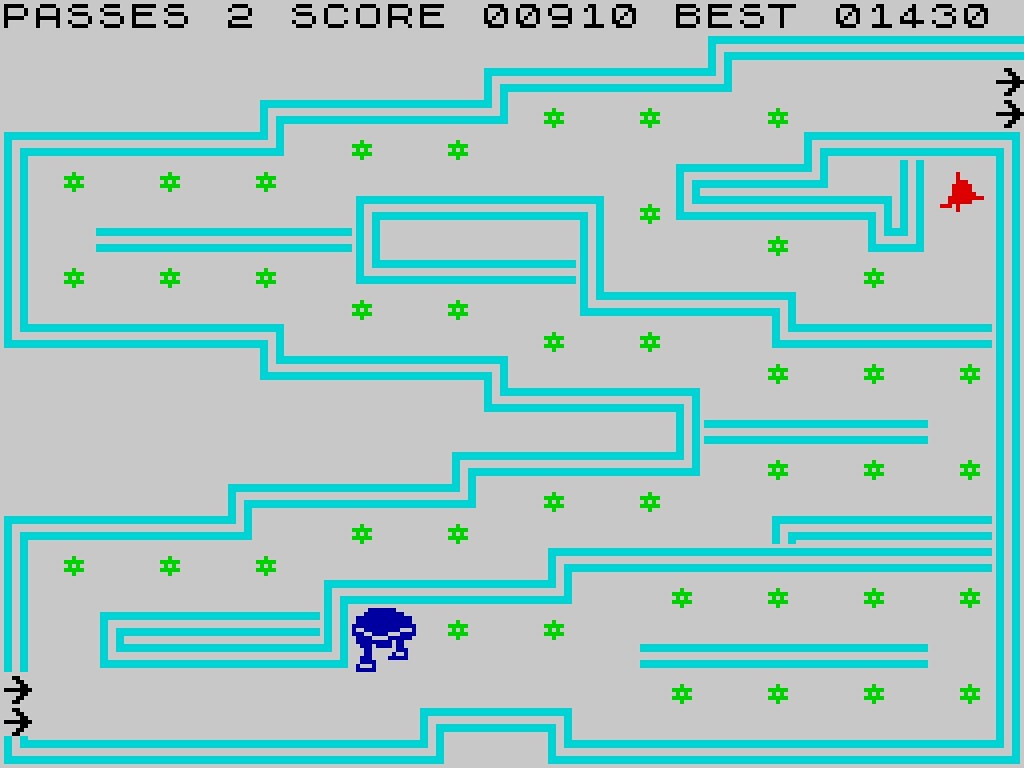This still image, designed in a nostalgic 8-bit pixel art style reminiscent of classic video games, showcases an intricate maze delineated by thin aqua blue lines. Within the confines of this labyrinthine structure, small, vibrant green star shapes are dispersed. In the center of the action, a round, purple character equipped with two legs navigates the maze, indicative of a player-controlled avatar. Nearby, a red triangular icon resembling a spaceship adds an element of urgency or pursuit to the scene. Dominating the top of the screen, the game interface provides crucial information: the current phase is labeled as "Phases 2", the player's score stands at "00910", while the best recorded score is "01430", setting the stage for the challenge at hand.